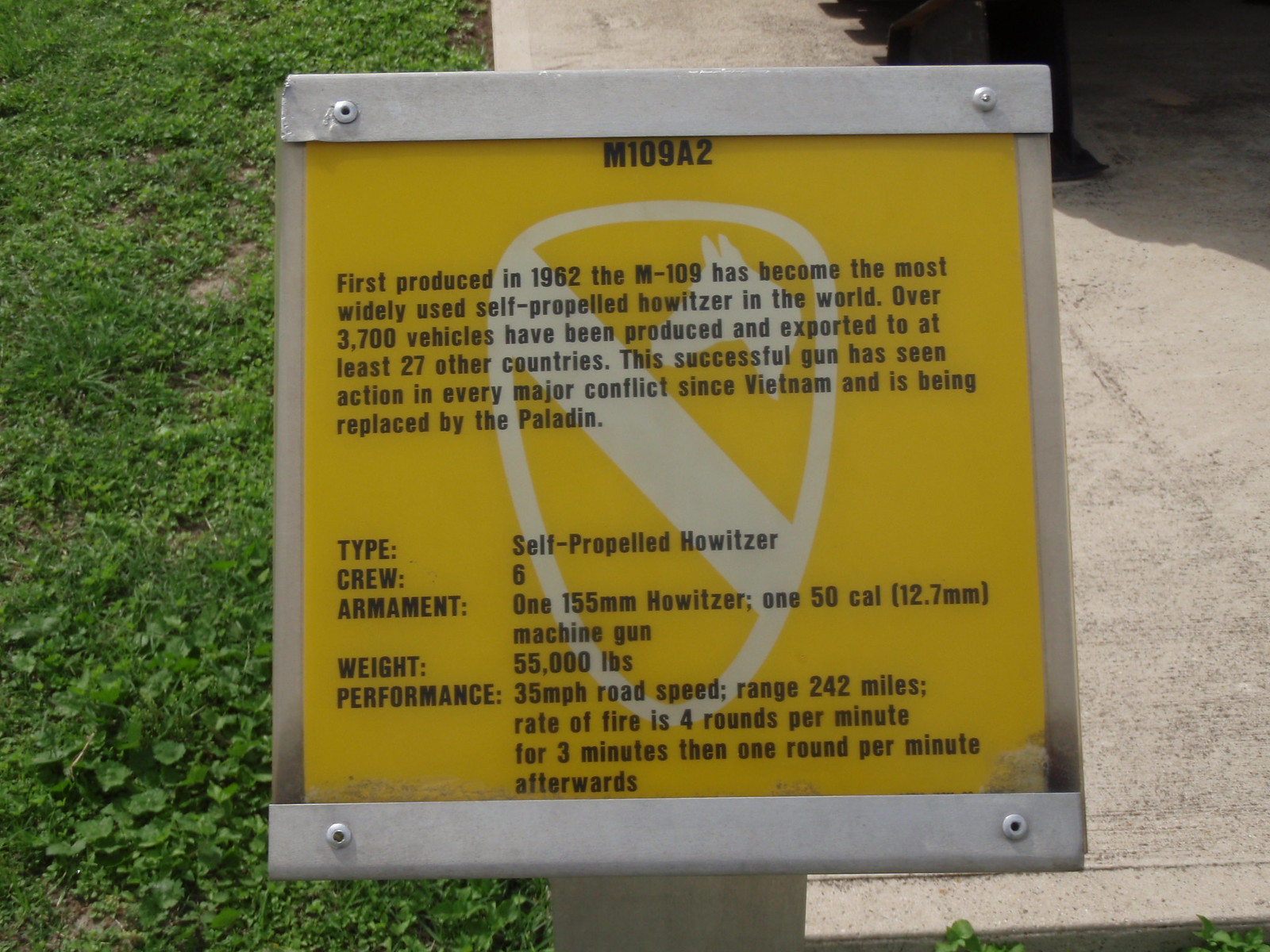In the foreground of the image, there is an informational placard mounted on a thick rectangular metal stand. The placard itself is set into a bolted metal frame and appears to be made of plastic or acrylic. It has a yellow background and displays a prominent white shield with a cross running from the top left to the bottom right of the shield, and a horse head situated in the upper right section of the shield. At the top of the placard, the text reads "M10982" in black letters. Beneath this, there is a detailed column of text that begins with "First produced in 1962, the M-109 has become the most widely used self-propelled howitzer in the world. Over 3,700 vehicles have been produced and exported to at least 27 other countries." More detailed specifications about the vehicle, including crew, armaments, weight (55,000 pounds), speed, and range, are also listed.

The setting is outdoors, with a manicured green lawn visible to the left of the placard and a concrete platform to the right. The metal frame holding the placard has large bent pieces of metal at the top and bottom and is secured by metallic pins on either side. The overall appearance suggests that the placard serves an educational purpose, possibly as part of a military showcase.